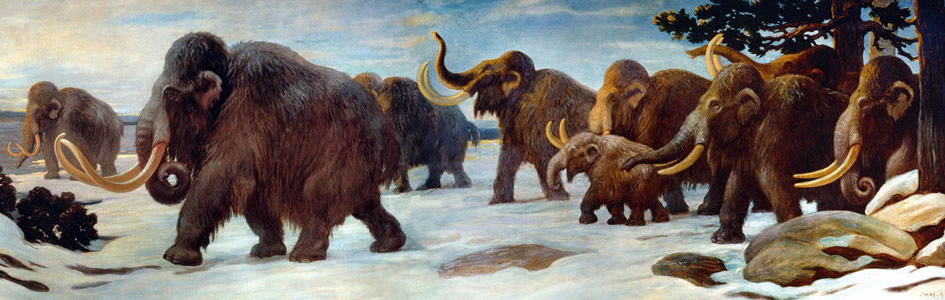This painting depicts an outdoor scene featuring a herd of approximately ten woolly mammoths traversing a snowy landscape during the daytime. Most of the animals are adults, characterized by their dense brown or black fur and impressive, curved tusks, which range in color from orange to brown. One of the notable mammoths has its trunk raised high, while the others have their heads lowered, seemingly focused on the snow beneath their feet.

A baby mammoth is protected between two adults, emphasizing the familial and social aspects of the herd. The mammoths are moving from the right to left across the canvas, creating a sense of motion. The snow-covered ground is interspersed with rocks, and in the top right-hand corner, a green-leafed tree provides a touch of vibrant color against the predominantly white and blue backdrop. 

The background features a clear blue sky with scattered white clouds, adding depth to the panoramic scene. This wide, rectangular painting captures the majesty of these prehistoric creatures in lifelike detail, from their textured fur to their gleaming tusks. A subtle detail in the center of the painting is a hole in the snow, possibly revealing water or frozen ice beneath.